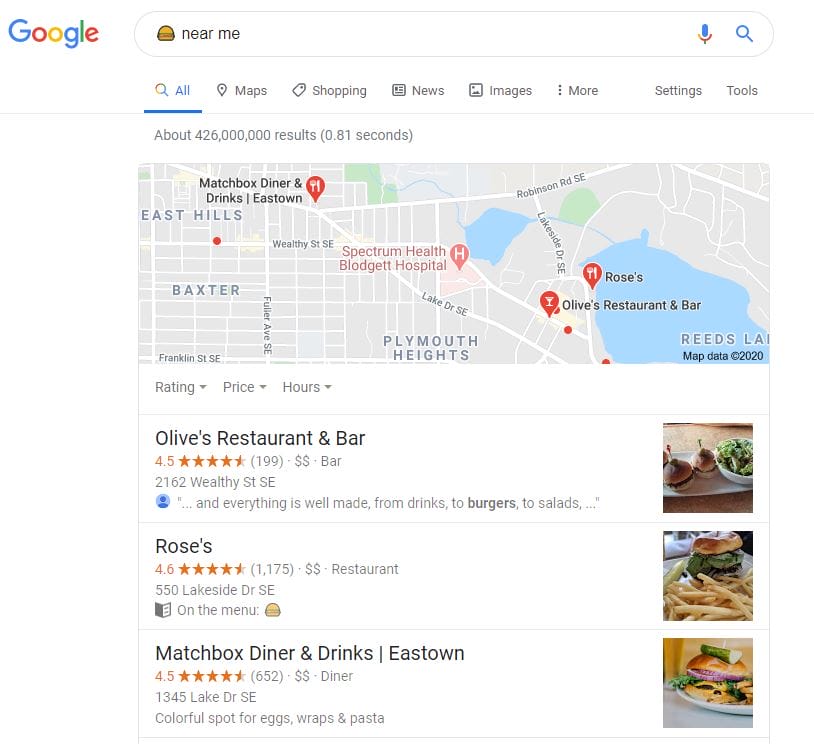In this image, the background is white, indicating it is a screenshot from Google. On the top left side, the recognizable Google logo is prominently displayed, featuring its characteristic blue, red, yellow, and green colors. Adjacent to the logo is a long, white search bar containing the black text "Near Me." To the left of this text is a hamburger emoji. Below the search bar, there are various tabs. The first tab on the left, labeled "All," is highlighted in blue text with a blue line underneath it. Following to the right, in light gray text, are additional tabs: "Maps," "Shopping," "News," "Images," "More." Further to the right, there are options labeled "Settings" and "Tools."

Below the "All" tab, there is a line of light gray text indicating "About 426 million results (0.81 seconds)." Underneath this line, a small Google map is displayed, featuring a network of thin, rectangular roads. In the center of the map, red text marks a location: "Spectrum Health Blodgett Hospital." Below the map, three restaurants are listed. The first is "Olives Restaurant Bar," marked with orange stars indicating a 4.5 rating. The second restaurant, "Roses," has a 4.6 star rating, and the third, "Matchbox Diner and Drinks, East Town," is rated 4.5 stars out of 5.